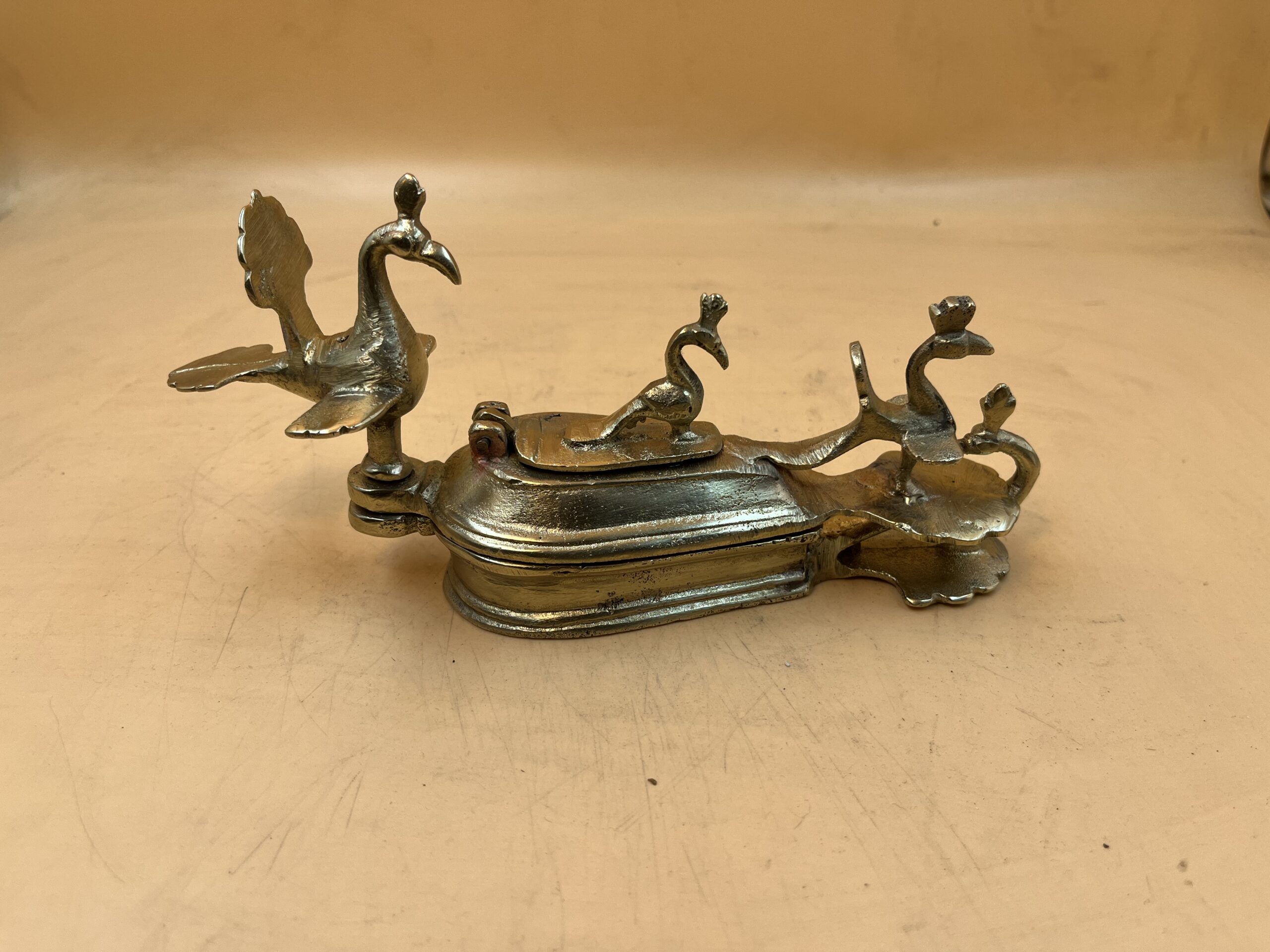A detailed bronze metal sculpture of three doves sits horizontally on a scratched yellow table, which extends into the background of the image. The sculpture, potentially a door knocker or an ornate decoration, features three distinct birds. On the far left, a bird perches delicately on a small post. In the middle, a smaller dove rests on an oval platform. To the far right, another bird, with its body and head turned rightward, faces forward. Below the entire piece, there is a rounded base. The table, or possibly a mat that has seen much use, is characterized by numerous scratch marks and adds a rugged yet nostalgic backdrop to this unique, heavy-looking metallic object.